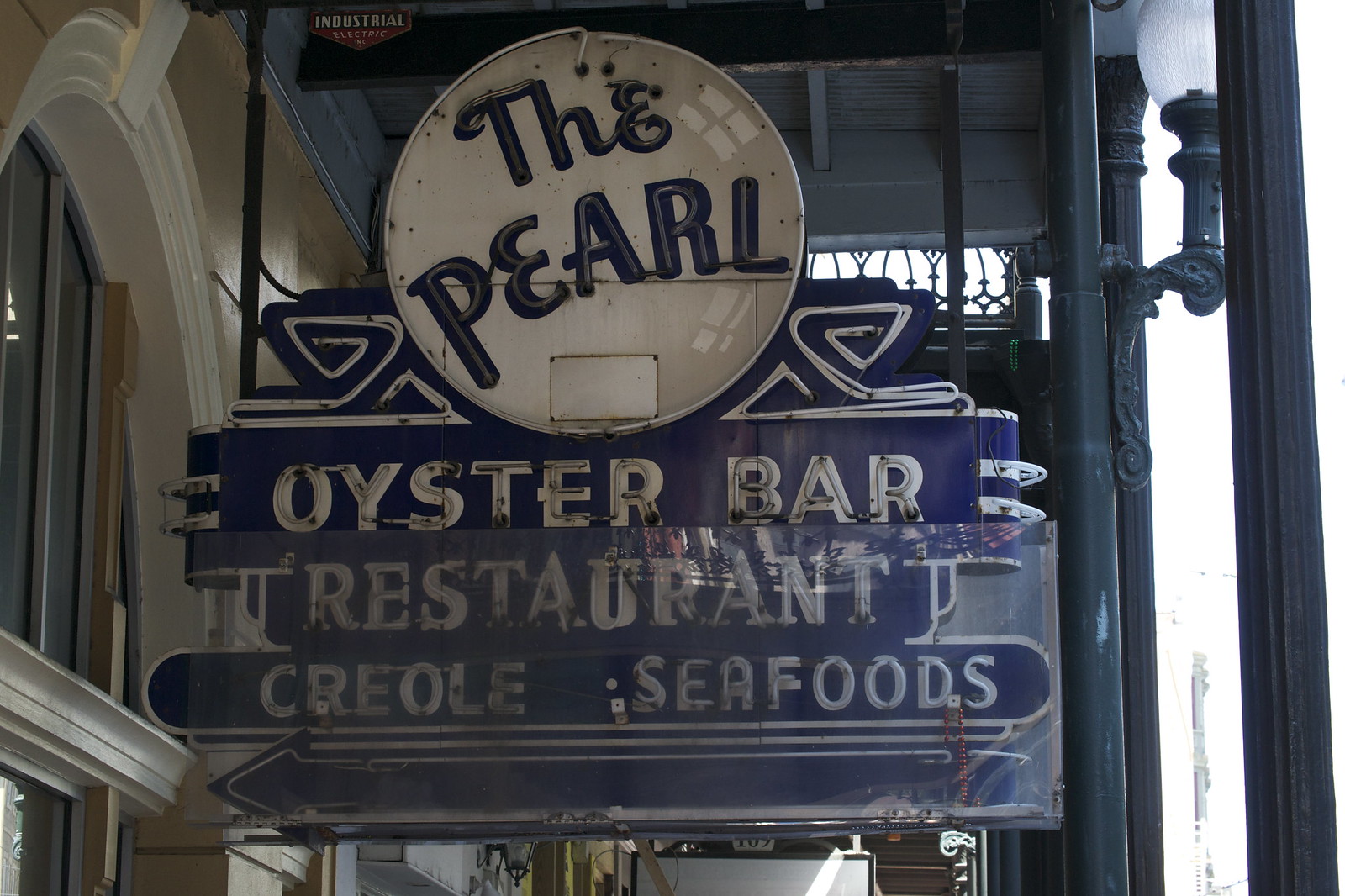The image showcases the exterior of "The Pearl" restaurant, prominently featuring a large, illuminated white circular sign with the establishment's name in black lettering, designed to resemble an actual pearl through detailed shading and lighting effects. Below the main sign, there is a blue banner with white text that reads "Oyster Bar," "Restaurant," and "Creole Seafoods," each phrase potentially illuminated by neon tubing designed to light up at night. The scene appears during the day and includes surrounding structural elements such as dark metal posts, including one with a multi-globe streetlight attachment on the right side. On the left, an arched window next to a glass door, possibly indicated by a blue arrow, suggests entry to the building. The setting, with its detailed signs and street elements, hints at a bustling location like New Orleans.